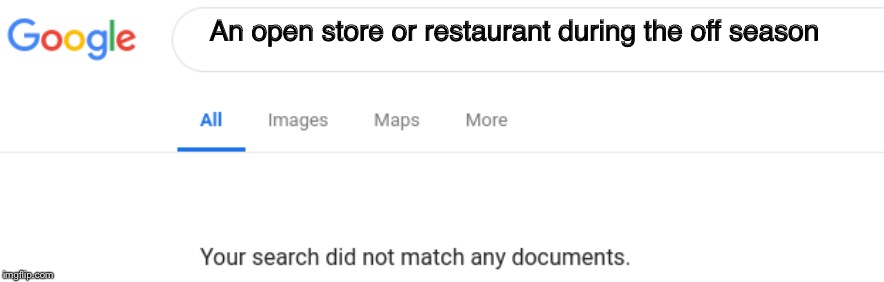This image captures a Google search results page where the query "an open store or restaurant during the off season" has been typed into the search bar. The familiar Google logo is prominently displayed at the top, with each letter in its characteristic color: the capital 'G' in blue, the first 'o' in red, the second 'o' in yellow, the lowercase 'g' in blue, the 'l' in green, and the 'e' in red. Below the search bar, the navigation options "All," "Images," "Maps," and "More" are visible, with the word "All" highlighted in blue, indicating the active tab. A thin gray line separates this header section from the search results below. The results area shows a message from imageflip.com on the left, stating "Your search did not match any documents" in the bottom right corner, indicating that no relevant results were found for the given search query. The overall design is clean and typical of Google's user interface, with a minimalistic and user-friendly layout.